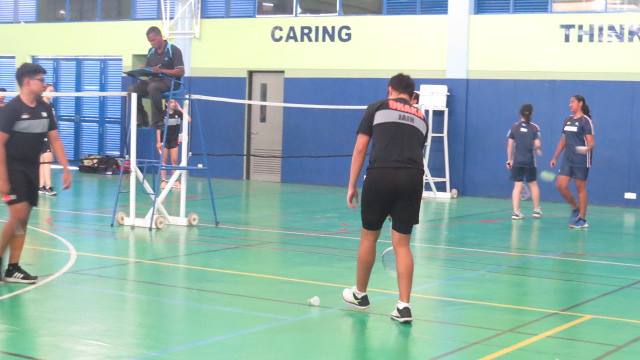The photograph captures an indoor gymnasium set up for both volleyball and badminton. In the center, there is a volleyball court equipped with nets and a high referee chair, approximately five or six feet tall, on a blue stand. The referee, dressed in a black shirt and black pants, holds a clipboard as he oversees the game. Six players, in identical black shirts and shorts with their names displayed on their backs, are preparing for play. A birdie lies on the green floor marked with various red, yellow, white, and black lines, hinting at an ongoing badminton game. Nearby, another team dressed in dark blue uniforms with white stripes on their shorts can be seen, suggesting that two different matches might be occurring simultaneously. The gymnasium’s backdrop features a mostly blue wall with a yellow strip at the top, characterized by a khaki-colored door, windows adorned with blue shades, and the words "Caring" and "Think" prominently displayed in English. This scene likely indicates an American setting.